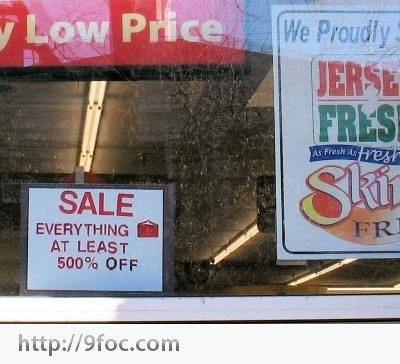This photograph captures the exterior window of a storefront, which appears dirty. The window features several signs, and beyond them, you can see the store's brightly lit ceiling with long fluorescent lights. Prominently displayed at the top is a red acrylic sign with white text that reads "Low Price." Below it, taped to the glass, is a smaller white sign with red print announcing a dramatic discount, "Sale. Everything at least 500% off." To the right, partially cropped by the edge of the image, is a multi-colored poster that reads, "We proudly" followed by "Jersey Fresh," and part of the phrase "as fresh as." The incomplete text also shows the letters "SKIN," suggesting it might say "Skinny Fries," although this is not certain. At the bottom of the image, a watermark is visible, providing the URL "http://9foc.com."